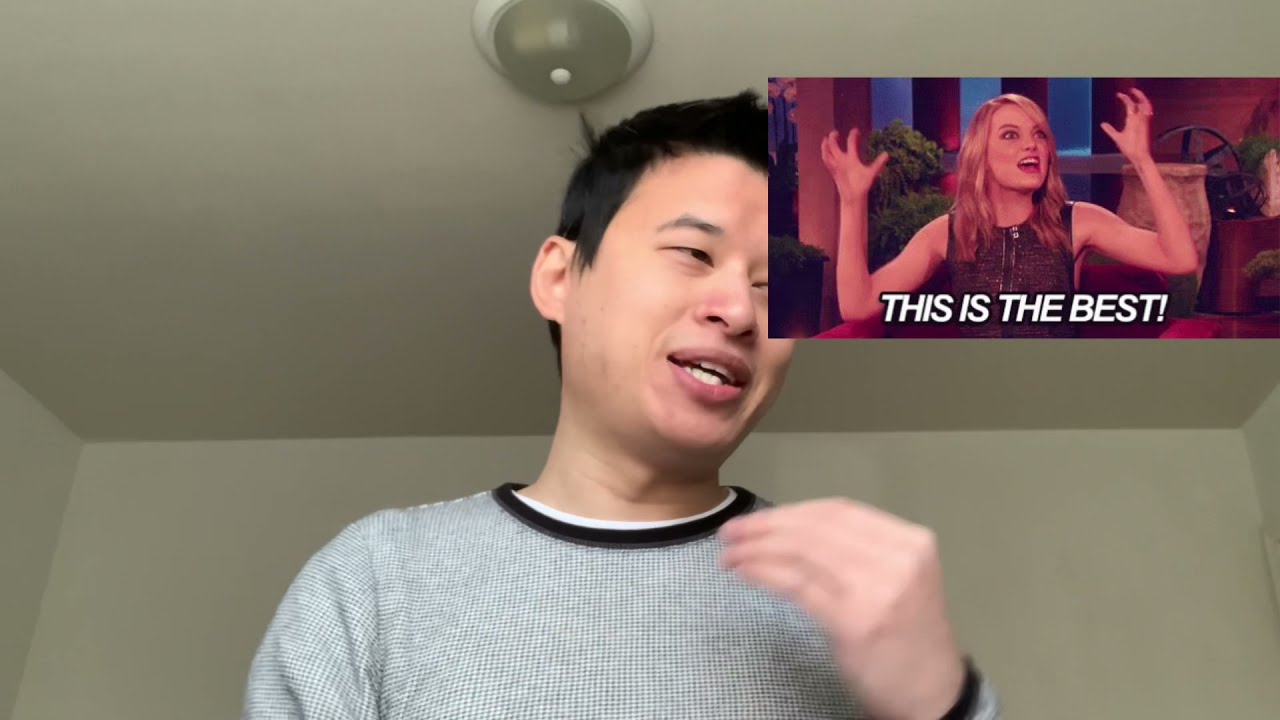The photograph captures a moment featuring two distinct subjects, one in the main frame and another in an inset image. The primary focus is on a man of Asian descent with short, dark hair, who appears to be in mid-conversation. He's wearing a gray waffle-knit shirt with black trim around the neckline and wrists over a white t-shirt. His left hand, slightly blurred, is positioned in front of him as if he's gesturing emphatically. He is looking down and to the right, with his mouth open, possibly speaking. The background reveals a light brown, unadorned wall and ceiling, with an unlit ceiling light.

In the top right corner of the main image is a smaller, inset image of a woman resembling Emma Stone. She has long, blonde hair cascading over her shoulders and is wearing a sleeveless, brown top, potentially with a front zipper. Her hands are raised, and she appears to be speaking loudly, her gaze directed upwards and to the right. The overlay text in white letters reads, "This is the best!" suggesting a lively expression. The background of her image hints at a studio setting with a beige vase and potted plants.